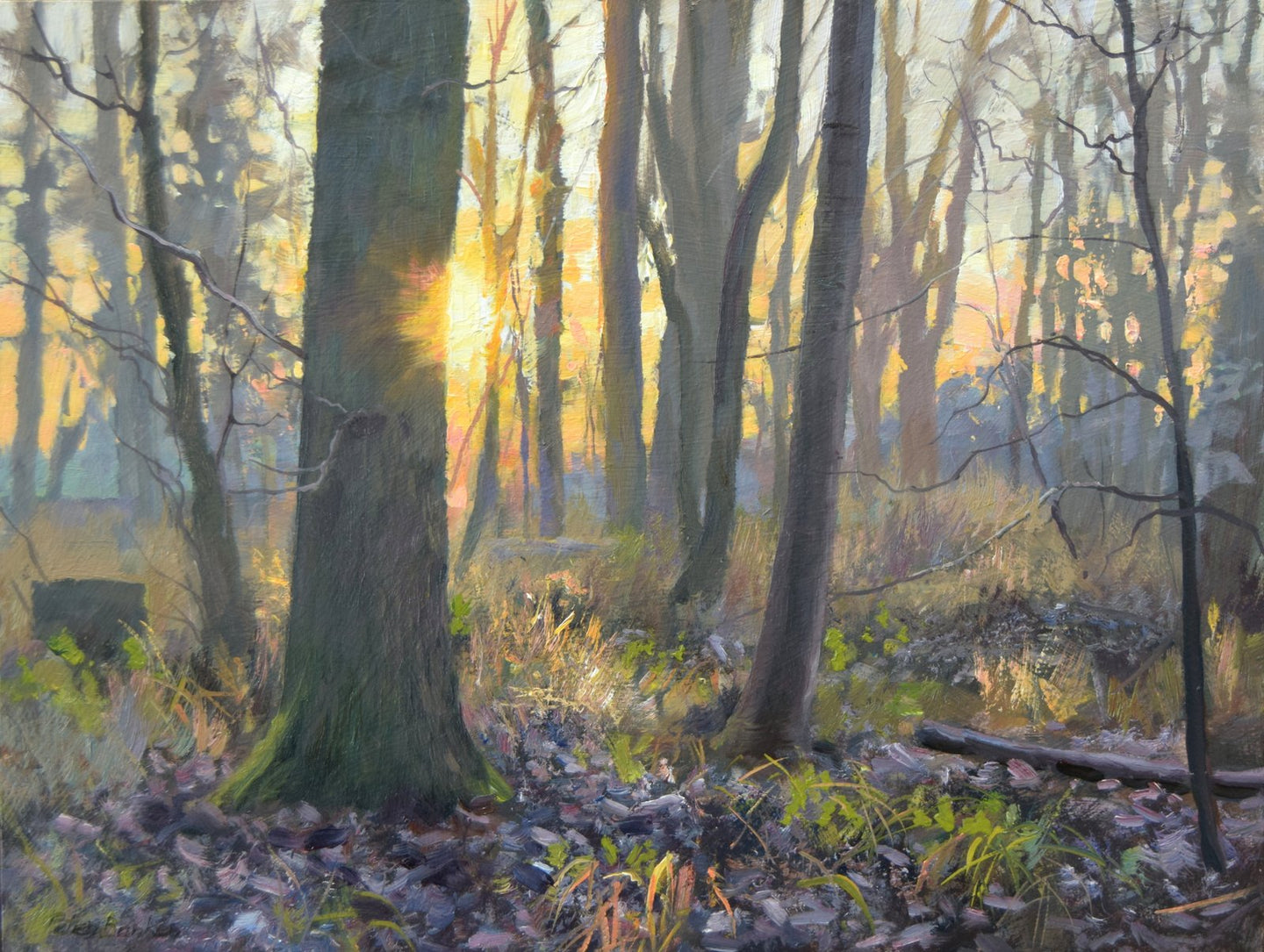This is an extremely detailed, full-color oil painting showcasing a dense forest scene in what appears to be fall or early spring. The square, borderless canvas vividly captures the natural light of the setting sun, which peeks through the many bare tree trunks and branches, creating a dramatic golden-yellow burst in the center-left of the image. The sky above transitions from a hazy blue near the horizon to a lighter blue at the top. The forest floor is scattered with dead leaves, sparse patches of brownish-green grass, and occasional grey rocks, giving a sense of the season. A fallen tree rests in the bottom left corner, adding depth and texture to the scene. Despite the density of the trees, the painting allows glimpses of the bright sky, enhancing the realism and depth of the outdoor setting. The craftsmanship is so meticulous that it could be easily mistaken for a photograph at a quick glance, attesting to the artist's skill. No people, animals, or artist's signature is present, focusing the viewer’s attention entirely on the beautifully rendered natural landscape.